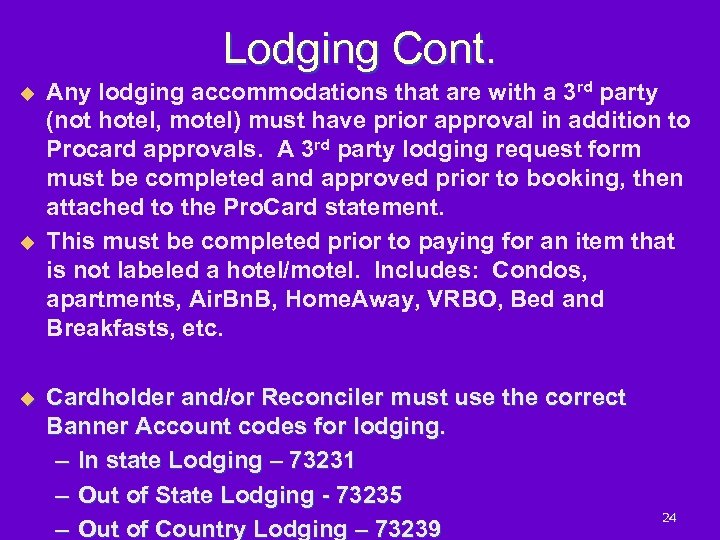The image features a bright purple background with a heading at the top that reads "Lodging C-O-N-T." Below this heading, there are three yellow, diamond-shaped bullet points. 

The first bullet point states that any lodging accommodations with third parties (not hotels or motels) require prior approval alongside ProCard approvals. This includes completing and approving a third-party lodging request form before booking and attaching it to the ProCard statement. 

The second bullet point emphasizes that this form must be completed prior to paying for lodging not categorized as a hotel or motel, which includes options like condos, apartments, Airbnb, HomeAway, VRBO, and bed and breakfasts.

The third bullet point specifies that the cardholder and/or reconciler must use the correct Banner account codes for lodging: 73231 for in-state, 73235 for out-of-state, and 73239 for out-of-country lodging. Additionally, the number "24" is located in the bottom right-hand corner of the image.